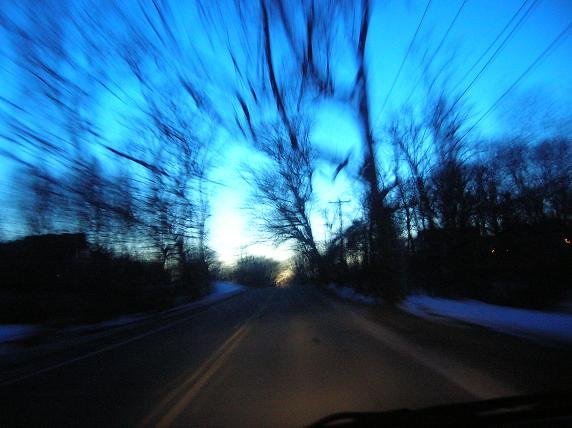A photograph captures the view from the front of a car through the windshield. The lower part of the image is partially obscured by the dashboard. The scene outside shows a road flanked by side rails, with the environment appearing somewhat blurred due to the car's motion. It is dusk, and the diminishing light casts a shadowy quality over the landscape. In the background, a line of buildings and trees is faintly visible, interspersed with numerous power lines and poles. The sky retains a hint of blue, though it's streaked with several indistinct black lines, likely from the shadows of passing tree limbs. The overall image conveys a sense of speed and the encroaching darkness of evening.